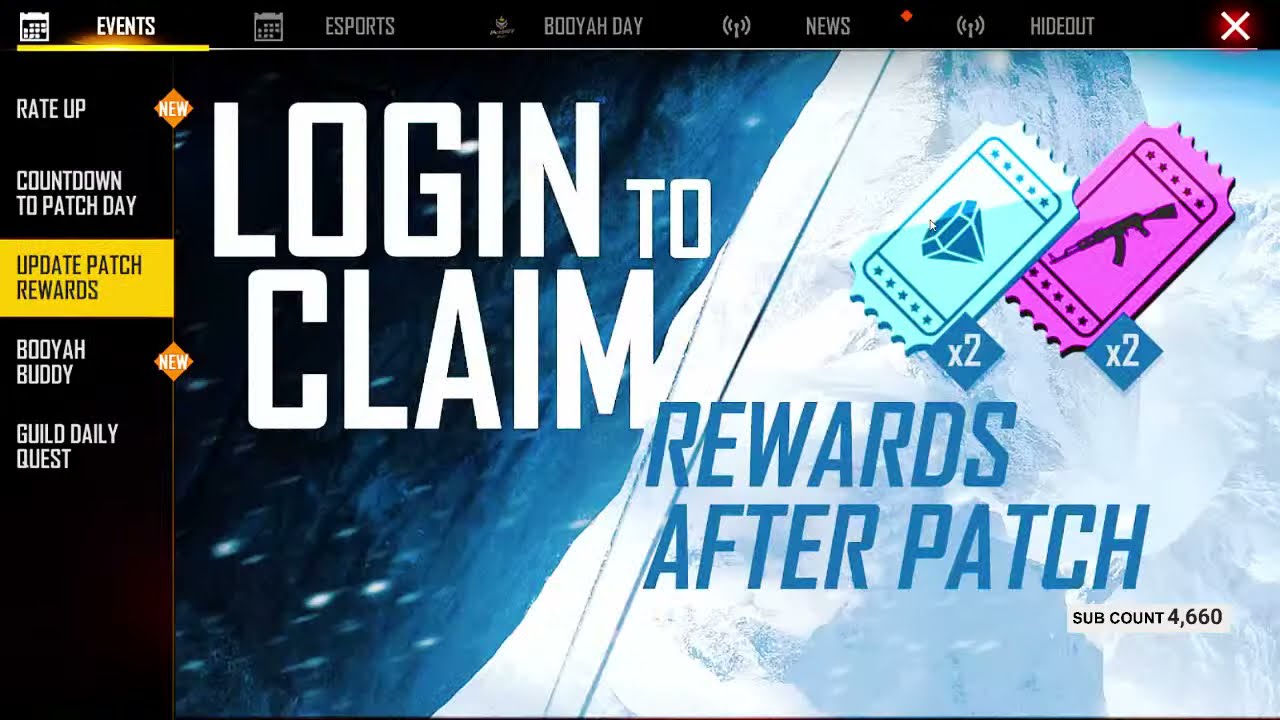This is a horizontal, rectangular screenshot from a video game's menu system. At the top, a solid black bar stretches from left to right, displaying tabs labeled "Events," "Esports," "Booyah Day," "News," and "Hideout." In the top right corner, there's a red 'X' for closing the menu. On the left side, a wider black border runs vertically containing several white text labels: "Rate Up," "Countdown to Patch Day," "Update Patch Rewards" (highlighted with a yellow rectangular background), "Booyah Buddy," and "Guild Daily Quest."

Dominating the center of the screen in large, all-caps white letters is the message "LOG IN TO CLAIM." Beneath this, in blue letters, it reads "Rewards After Patch." The background behind these texts is blue. On the upper right section of the image, there are two tickets: a light blue one with a gem in the middle and a label "x2," and a purple one featuring a rifle, also with a "x2" label. The area behind these tickets has a silver and light blue background, resembling the side of a mountain with the sky just visible in the top corner.